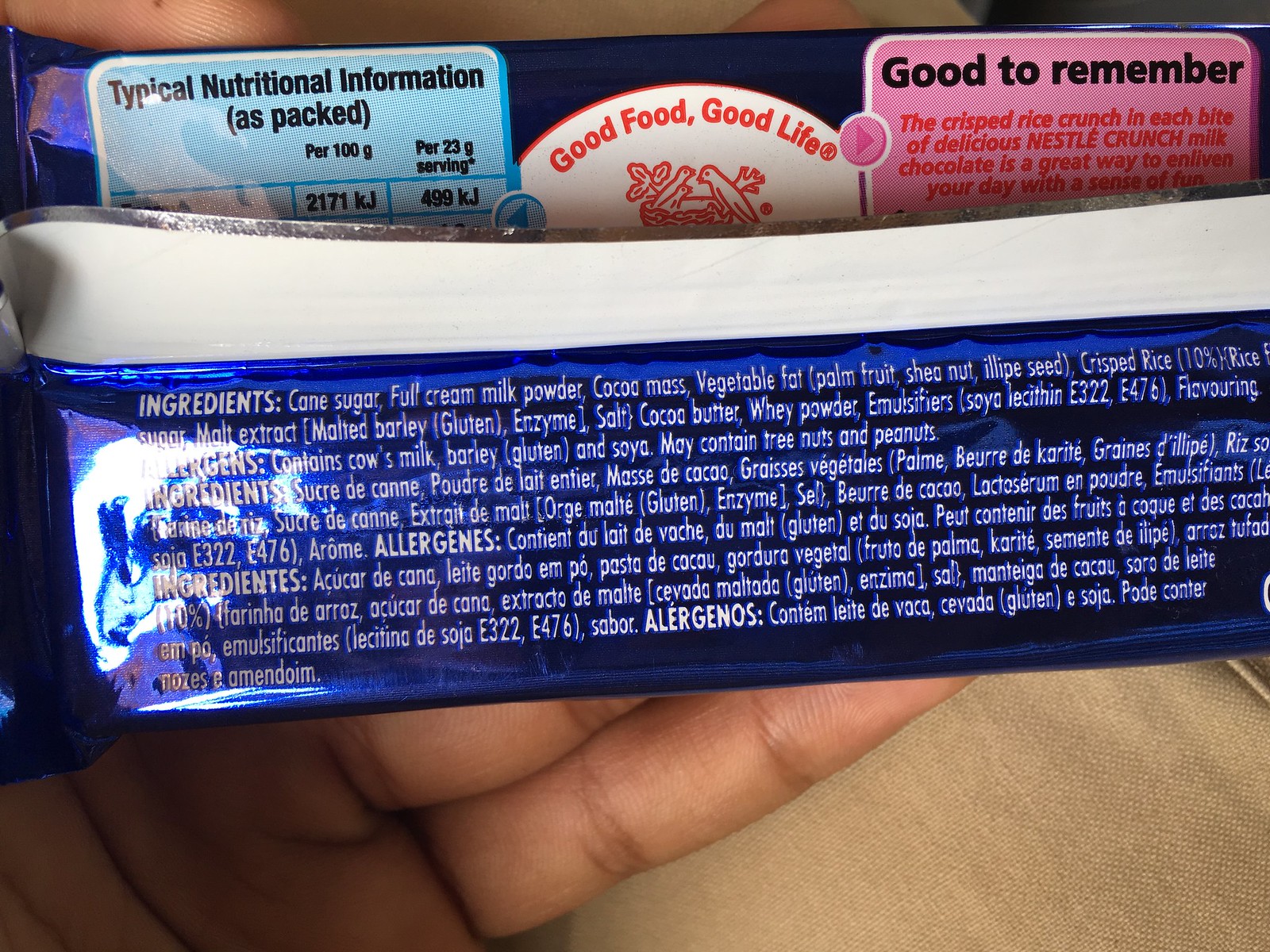The image features the backside of a Nestlé Crunch bar, wrapped in distinctive blue foil. At the top left, a blue rectangular box provides nutritional information, accompanied by the caption "Typical Nutrition Information Is Packaged." On the opposite side, a pink rectangular box bears the message: "Good to Remember: The crisp rice crunch in each bite of delicious Nestlé Crunch milk chocolate is a great way to enliven your day with a sense of fun. What is Nestlé Crunch?"

Centrally positioned and slightly cropped from view, there is a logo of a white half-circle outlined in red. Within this logo, the text reads "Good Food, Good Life," alongside an illustration of three birds nestled in a cozy nest. The lower half of the packaging displays detailed nutritional facts, emphasizing the commitment to transparency about the contents of this iconic chocolate treat.